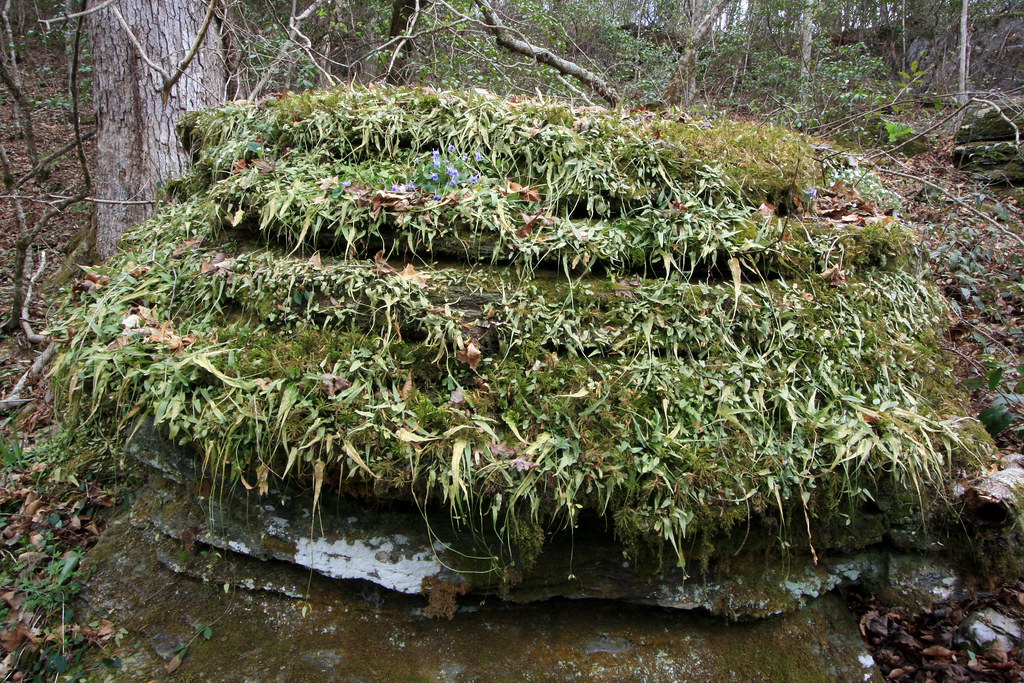This picture captures a serene woodland scene, likely set in the mountains during the day. The focal point is a unique, rectangular rock structure that appears stepped or staged in various levels, covered with lush green irises or lilies interspersed with moss and perhaps some ferns. Among the rocks and foliage, overgrown grass and brown leaves add a natural, untouched feel to the setting. In the background, tall tree trunks rise up, adding depth to the scene. The entire structure is enveloped by dense moss, suggesting it has been there for some time, blending seamlessly into its forest surroundings. The natural lighting accentuates the vibrant greenery and the rich earthy tones, creating a picturesque woodland garden.